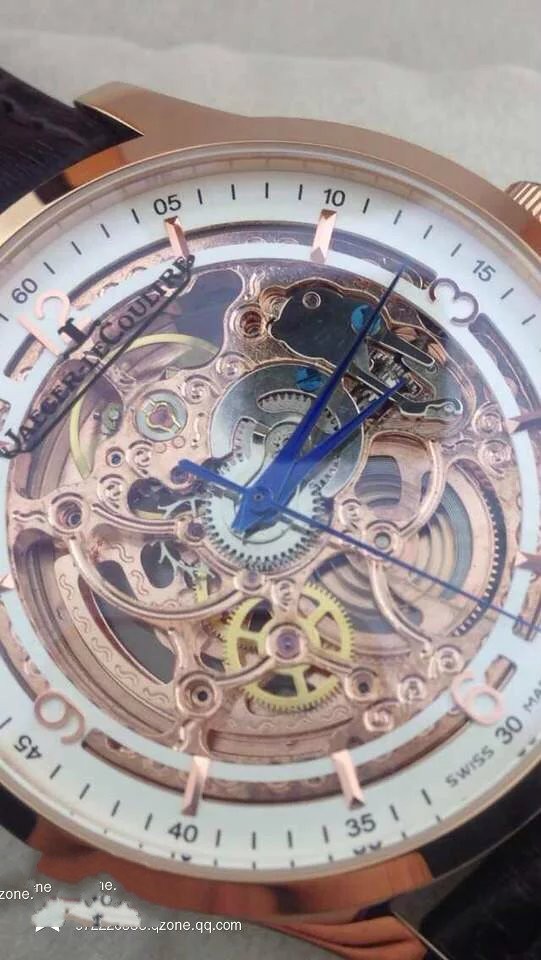This close-up photograph showcases an intricate wristwatch, highlighted by its sleek black leather band. The watch's bezel is elegantly crafted in a luxurious rose gold or brass tone. Surrounding the outer edge is a white ring featuring finely detailed second markers, calibrated up to 60 seconds, with precise tick marks encircling the dial. Prominently displayed brass numerals indicate 12, 3, 6, and 9 o'clock positions, complemented by major minute markers at 5-minute intervals.

The centerpiece of this timepiece is its transparent inner mechanism, revealing a captivating array of gears in silver, bronze, and gold hues. The watch hands are meticulously crafted, with the short hour hand pointing just past 3, the longer minute hand situated precisely at the 13-minute mark, and the second hand positioned around the 27-second mark. Adding a touch of sophistication, the name "UAEGER-LE COULTRE" is delicately inscribed on the face of the watch, encapsulating both elegance and engineering marvel.